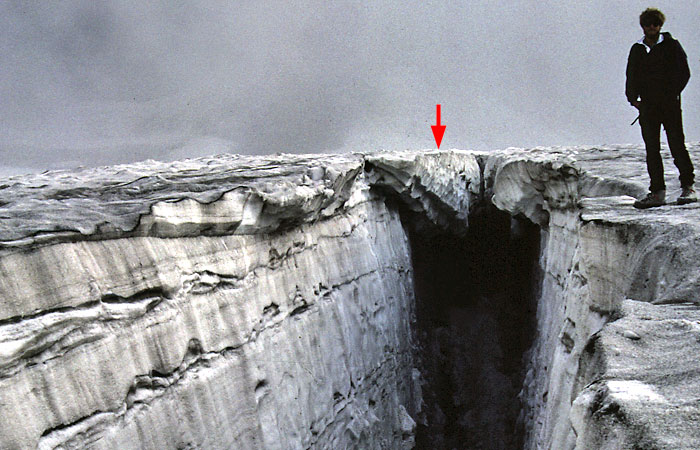In this wide rectangular photograph taken in an arctic or mountainous environment, a silhouetted man stands on a gray, jagged rock surface at the top right corner. He is dressed in a dark long sleeve shirt, dark pants, and boots, with curly hair partially visible. The man stands precariously on the ledge of a deep, steep crevice that cuts through the middle of the scene, which appears to be part of a glacier or mountain valley. The snow covering the crevice and the surrounding rock surfaces is discolored with gray, possibly due to environmental pollution. A vivid red arrow is drawn over the image, pointing to the left side of the crevice, where the rocky cliffs seemingly meet in the distance. The sky above is overcast with a dull gray hue, adding to the dramatic and somewhat desolate atmosphere of the photograph.